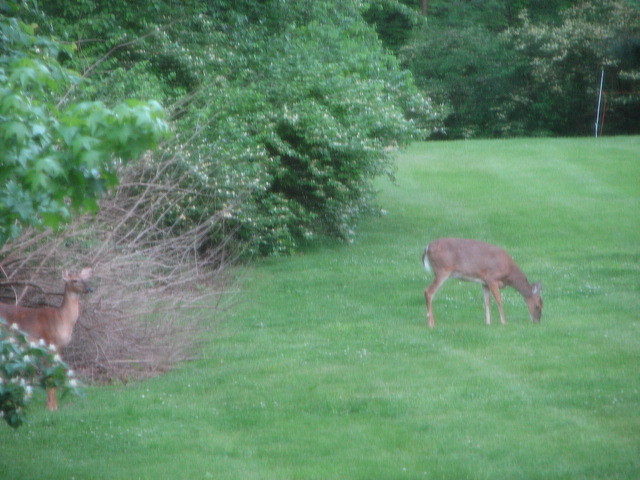This photograph captures a tranquil scene of two deer in what appears to be a lush, green backyard. One deer is bent down, intently grazing on the thick, vibrant grass that blankets the ground. The greenery is uninterrupted by dirt or rocks, suggesting a well-maintained area. Surrounding the field are dense clusters of bushes and trees, giving the space a forest-like feel. Among the predominantly green foliage, a single brown, desert-like tree or bush stands out.

The second deer, positioned towards the left side of the image, has a more cautious demeanor. It seems to be hiding partially behind the bushes, standing in a brown patch of brush and leaves, which contrasts with the overwhelming greenery of its surroundings. Both deer exhibit a rich brown coat with touches of white. 

Although the photograph is slightly blurred, it still emphasizes the lush, green ambiance of the setting, indicating a time of year when nature is fully in bloom. There are no human figures or text within the image, further highlighting the serene encounter with these shy creatures in their natural environment.